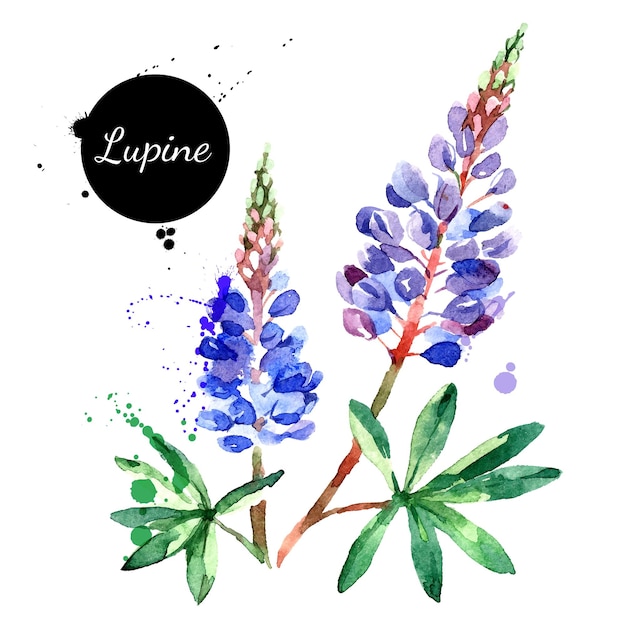This is a detailed watercolor painting of lupine flowers. At the top left, a black circle contains the word "lupine" in white cursive script. The artwork prominently features two lupine plants. Each plant has a distinctive pine cone-shaped inflorescence composed of multi-colored petals in shades of blue, purple, and red, with some green tips. The stems are reddish-brown, adorned with vibrant purple petals that ascend from the base. At the base of the plants are leaves that resemble seven-fingered hands, each consisting of an array of seven smaller leaflets in varying shades of green. Background details include subtle white paint splotches that add a textured depth to the scene.